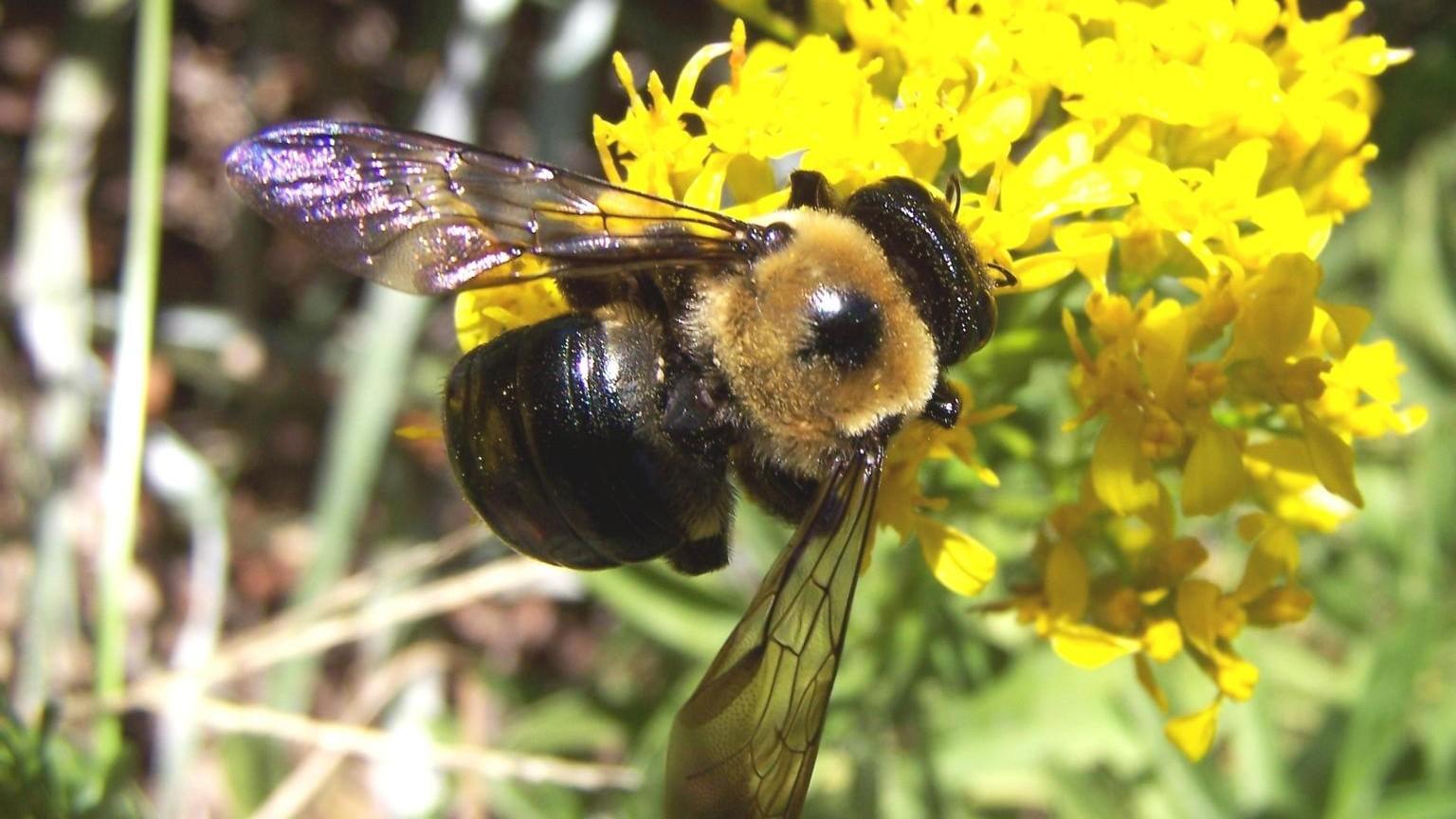This detailed close-up photograph captures a bumblebee amidst a wild outdoor setting, showcasing its meticulous foraging on a vibrant yellow flower under a bright sunlit sky. The bee, positioned diagonally, has distinct black and tan patterns. Its large, black abdomen and head exhibit smooth black surfaces with white highlights from the sunlight. The translucent wings, showing a hint of iridescent purples and blues, have noticeable black and skinny outlines within. The backdrop is filled with slightly blurred green grass on the right and tan weeds on the left, contributing to a chaotic yet natural landscape. The bumblebee, surrounded by a cluster of yellow flowers, collects pollen as the sunlight enhances the details, including some purple highlights likely due to lens aberrations, reflecting the vibrant essence of this outdoor moment.